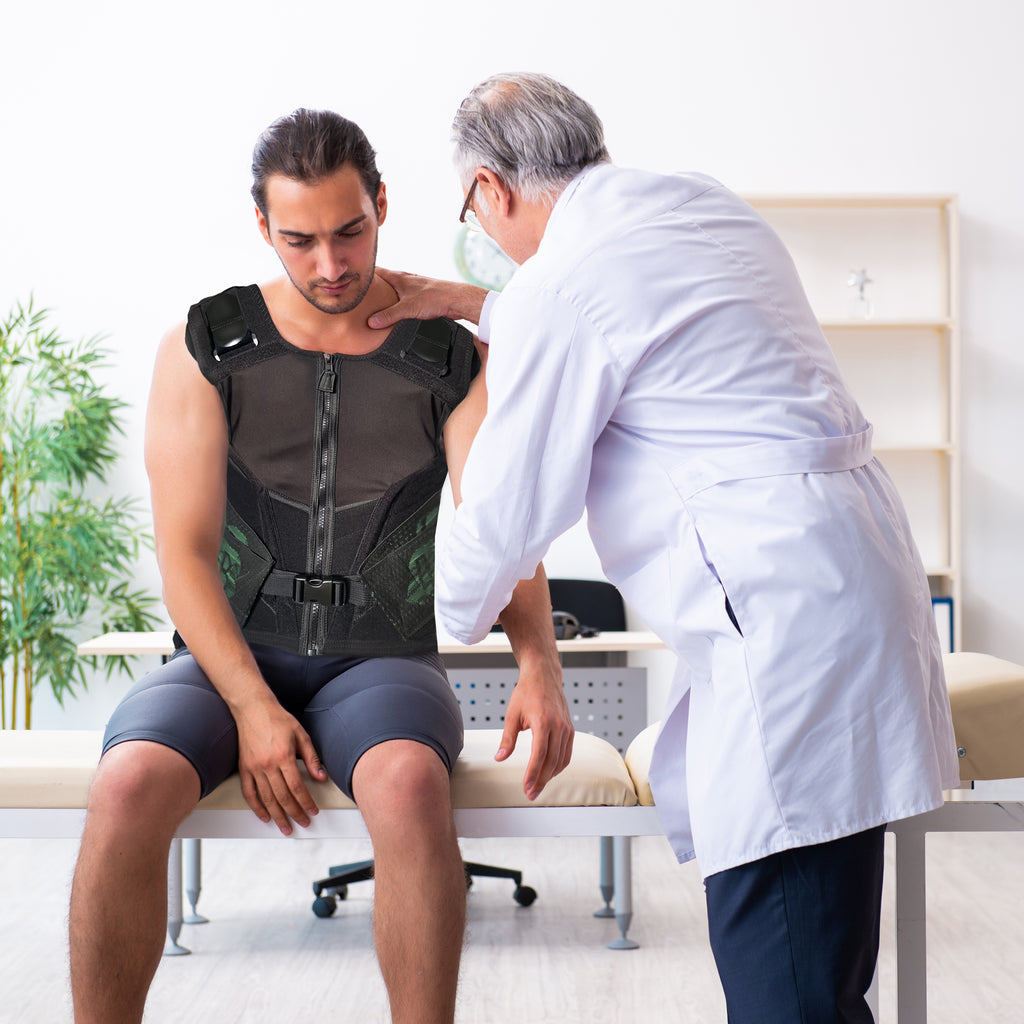In a bright, modern doctor's office, a man sits on a white-framed bench with a beige cushion, wearing a black vest with a center zipper and clip strap, along with blue compression shorts. His head is slightly lowered, suggesting discomfort. An older Caucasian doctor in a white medical coat, wearing glasses, stands to his right, examining the man's neck, shoulder, and left arm. The office features a doctor's desk, a computer, a clock on the wall, and a bookshelf. A green palm tree plant adds a touch of nature to the left side of the image.